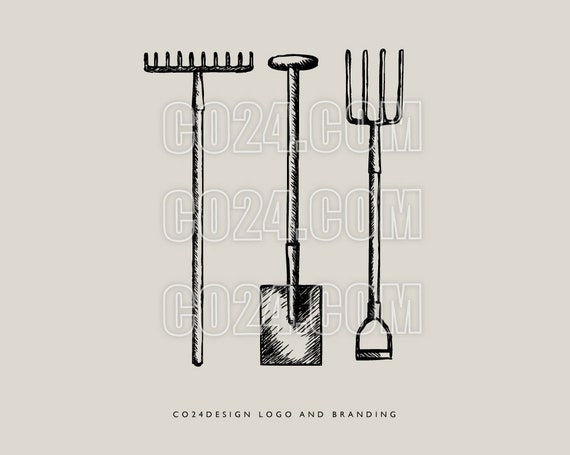The image is a rectangular poster with a light brownish-gray background. At the center, there is a transparent watermark featuring "CO24.com" repeated three times in white, vertical alignment. At the bottom, the text "CO24 Design Logo and Branding" appears in black. Displayed in the middle of the graphic are three outdoor tools: a wooden rake with a metal head on the left, a dark red flat shovel standing on its blade in the center, and a pitchfork with an open handle and upward-pointing tines on the right. The entire composition is rendered in black and white, except for the shovel, emphasizing the tools against the muted background.